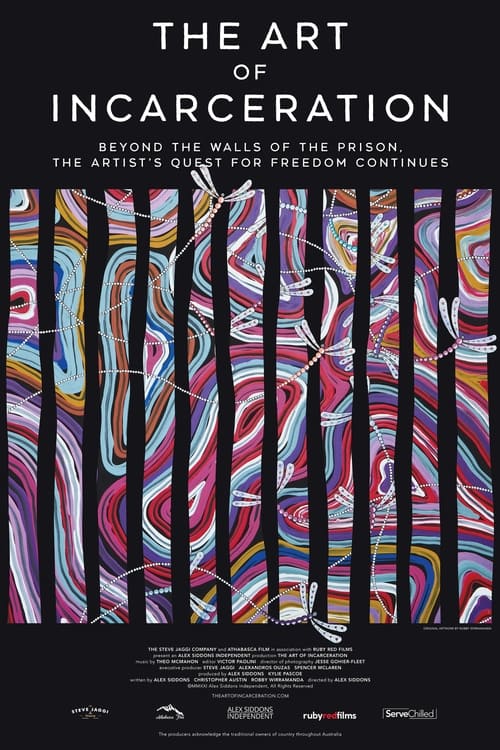This detailed poster, titled "The Art of Incarceration," features the phrase "Beyond the walls of the prison, the artist's quest for freedom continues" in white text against a black background. The title itself is prominently displayed, divided into three rows with "The Art" at the top, "Of" in the middle, and "Incarceration" at the bottom. Below this title, the vibrant and abstract art is showcased, featuring clusters of dragonflies amidst vertical, wiggly black bars that give a sense of confinement. Behind the bars, the background bursts with abstract, plant cell-like circles in a myriad of colors including green, blue, orange, pink, and purple, set against a deep black backdrop. Along the bottom edge of the poster, small white text details the credits, accompanied by five logos from various sponsors or contributors. The poster is further labeled with "Alex Siddon's independent ruby red films, serve chilled" at the very bottom.